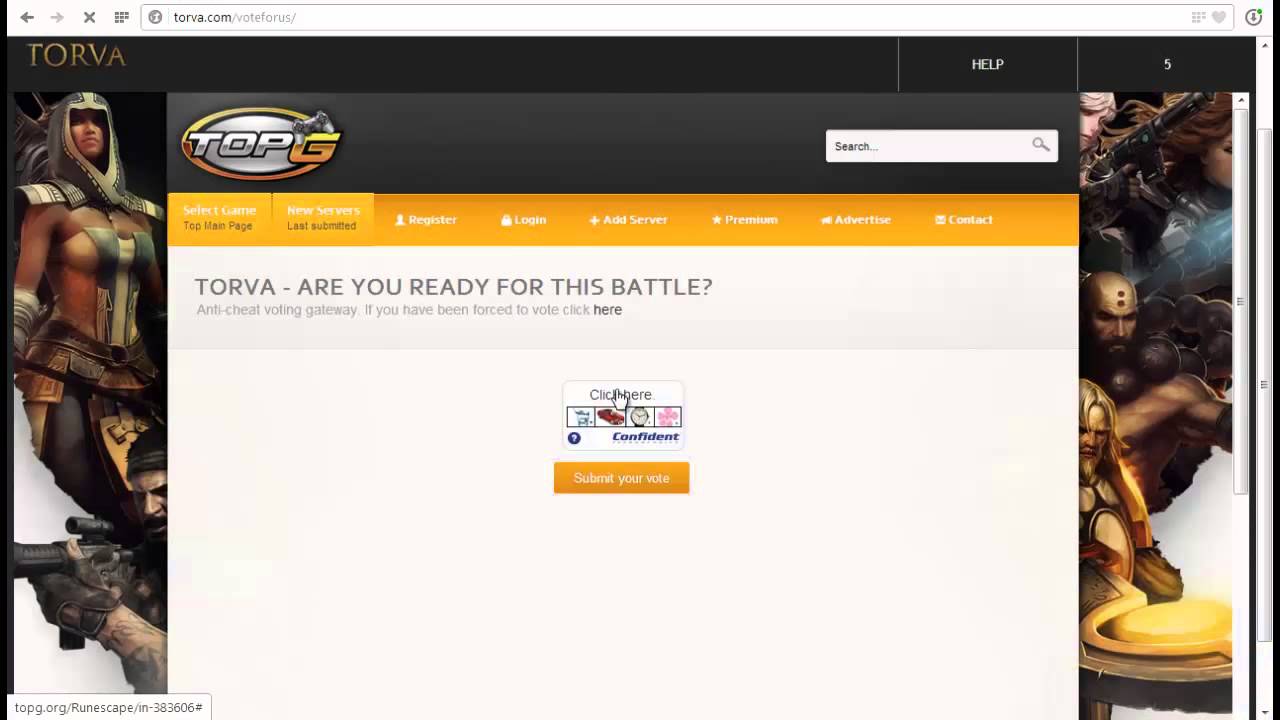In the image, we see a dynamic background featuring various action figures, including a prominent figure named Torva. The top portion of the image displays a website address, and there is a black rectangle with the word "help" on it, alongside another black rectangle containing the number 5. To the right, two scroll bars are visible.

At the top center, there is a search bar with placeholder text "search..." next to a magnifying glass icon. Adjacent to the search bar, a gray circle with the text "Top G" is present, where the "G" is highlighted in gold.

A bold headline reads, "Torva. Are you ready for this battle?", setting an adventurous tone. Below the headline, a vibrant orange rectangle features options to "Register" and "Log In". Additional interactive options like "Add Server," "Premium," "Advertise," and "Contact" are listed nearby.

There is also a call-to-action button in an orange rectangle stating "Submit Your Vote". Finally, at the bottom left corner, there's another rectangle containing a website address, reinforcing the connectivity and interactive elements of the image.